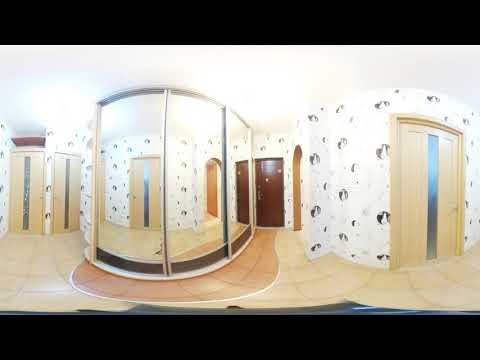The image captures the inside of a somewhat surreal, funhouse-esque space, likely a private home, depicted with a fisheye lens that creates a distorted, 360-degree effect. The space is marked by multiple doorways—three cream-colored ones to the left, a brown door possibly leading to a bedroom or bathroom beside a curved wall lined entirely with mirrors, and what seems to be entryways under arched designs to the right—suggesting it might be a lobby or hallway. The flooring is a mixture of cream and burnt orange stone tiles, and the walls are adorned with white wallpaper patterned with scattered black designs. The overall washed-out quality of the image and its odd angles give it an almost illustration-like appearance, making the environment appear peculiarly expansive and foreign.